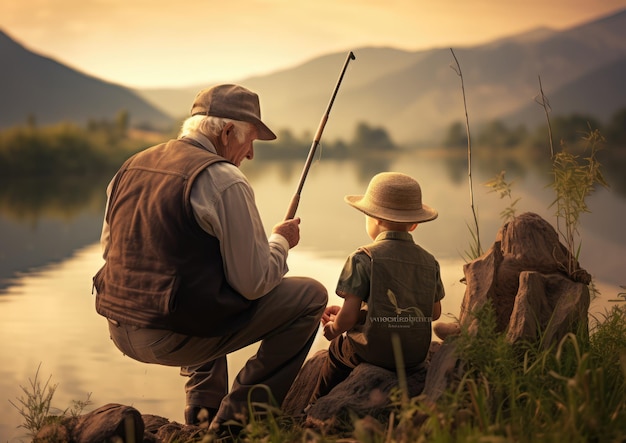A heartwarming, professionally captured photograph shows a grandfather fishing with his grandson. The grandfather, dressed in a brown vest, brown pants, a light tan long-sleeve shirt, and a brown hat, is kneeling down and holding a fishing pole in his left hand, gazing fondly at his grandson. The grandson, wearing brown pants, a green shirt, and a tan bolo-style hat, is sitting on a rock next to his grandfather, attentively listening. Beside the boy, there is a large rock formation. The scene has a picturesque background featuring a vast lake extending into the distance, where muted earth tones of browns, greens, and tans blend beautifully. Trees and bushes surround the lake, and a majestic blurred mountain range completes the tranquil setting.